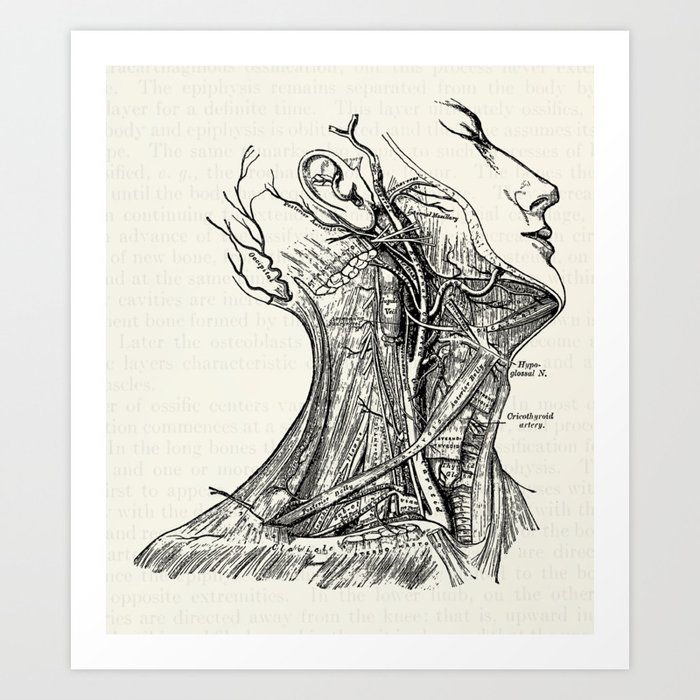This detailed black-and-white hand-drawn scientific illustration depicts a side profile of a human head and neck, meticulously rendering the intricate network of veins, arteries, nerves, and capillaries. The illustration showcases the anatomy from just above the eyebrows, excluding the forehead and hair, down to the base of the neck where it meets the shoulders. The human figure is shown with closed eyes, looking to the right, and includes detailed features of the nose, lips, chin, and right ear. The artwork extends to the jawline, back of the head, and collarbone area. The veins and nerves are prominently displayed, with accompanying text labeling various elements, though the text is somewhat obscured and difficult to read. The shading technique enhances the portrayal of muscle tone and density, lending a lifelike quality to the anatomical structures. The sketch is framed by a white border on a tannish-yellow background, adding a vintage scientific aesthetic to the piece.